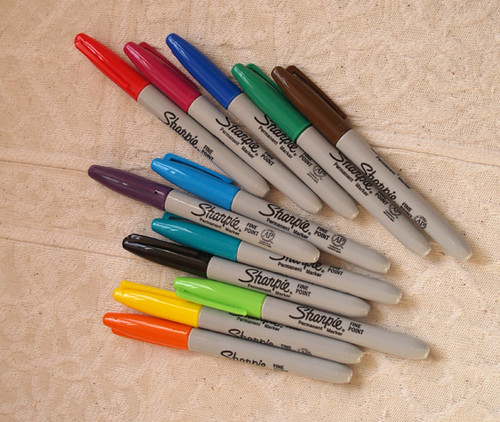The image displays a close-up, colorful photograph showcasing 12 fine tip Sharpie permanent markers, arranged haphazardly on a textured, cream-toned fabric background with an embossed, floral design. The markers lie almost side by side, starting at the bottom with seven of them slightly tilted toward the upper left corner and the remaining five at a steeper angle in the same direction. Each Sharpie has a gray body with caps in the following sequence from bottom to top: orange, yellow, pale green, black, turquoise, dark blue, sky blue, red, maroon, regular blue, forest green, and brown. The detailed background and the vivid caps create a striking contrast, emphasizing the array of colors and the texture beneath.